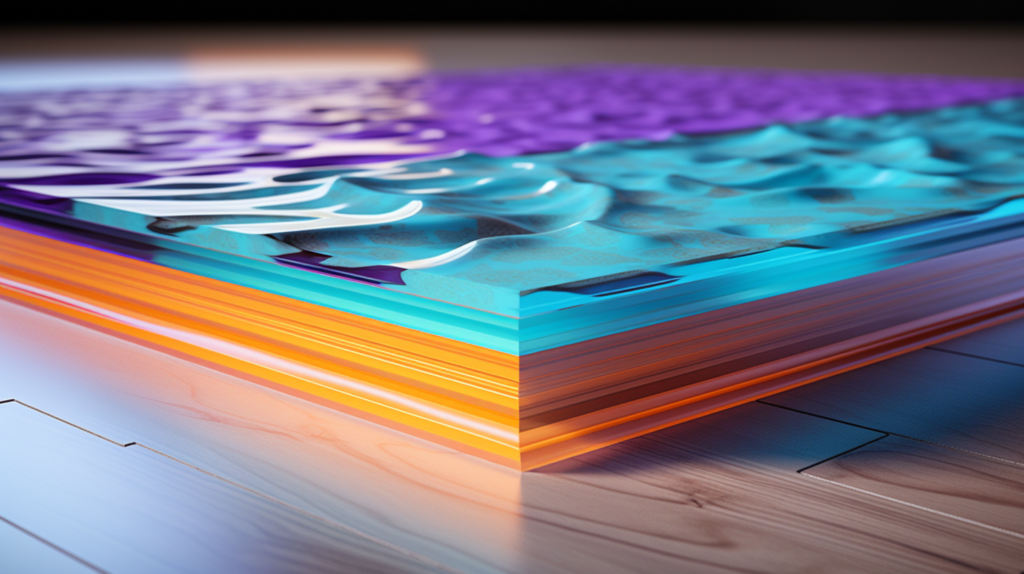In this computer-generated, abstract image set in landscape orientation, a structure consisting of layered, paper-like materials sits atop a hardwood floor. The hardwood floor, visible at the bottom left and right corners, is light in color and its planks fit together seamlessly. Rising from this floor is a square, box-like object characterized by its vivid and varied color palette. Central to the composition, the lower layers of the structure feature hues of orange, yellow, light brown, and cream, arranged in distinct strata. Above these, the top section of the object transitions to a clear, wave-like formation with blue and purple tones, resembling the ocean. The turquoise layer, punctuated with wave patterns, gives way to a purple segment, enhancing the sense of depth and dimension within this abstract, vividly colored design.